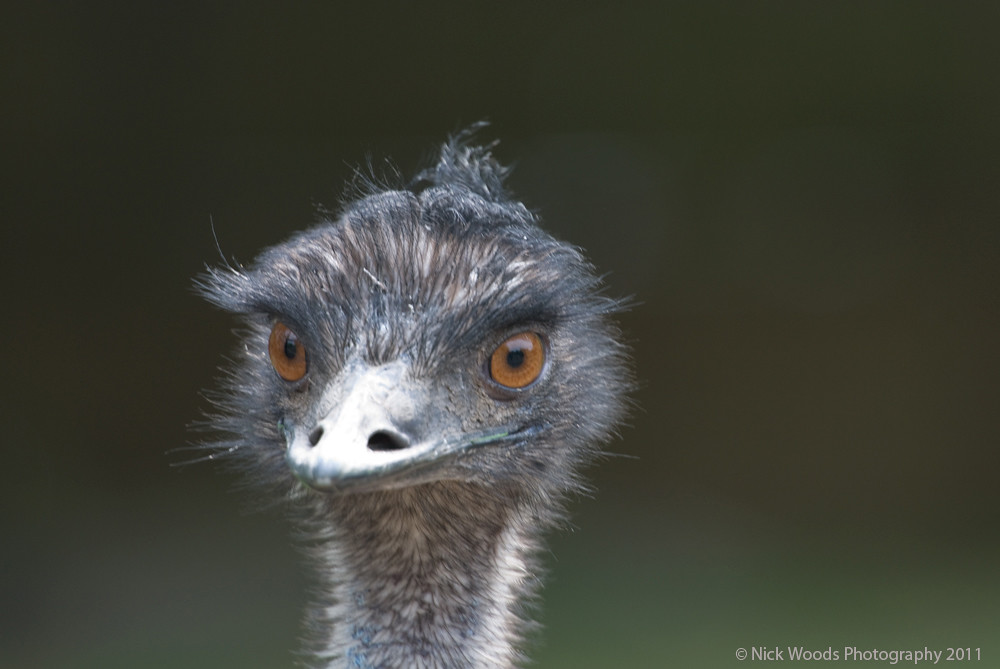This detailed headshot captures a close-up of an emu, set against a muted deep green-gray background that transitions to a dark green towards the bottom. The emu's neck extends upward from the bottom of the frame, leading to its uniquely shaped head, which appears almost like a small knob atop its elongated neck. The bird is looking slightly off to the left of the camera's focus, its beady eyes dominated by brown irises with stark black pupils. 

Its beak, silver-gray in hue and adorned with fairly large nostrils, almost appears white in the light. The emu's skin features a gray fuzz that reveals a speckled, soft white undercoat, extending from the top of its head down through its neck. Sprouting from the top of its head is a tiny wisp of hair, adding a whimsical touch to its appearance.

The emu's bushy, gray eyebrows and fine, gray feathers contribute to its distinctive look, which some might compare to a baby ostrich. In the lower right corner of the photograph, the caption "Nick Woods Photography 2011" affirms its authenticity and artistic origin. The bird's reflective eyes and the warm, textured details of its feathers stand out vividly against the muted backdrop, creating a compelling and intimate portrait of this fascinating creature.